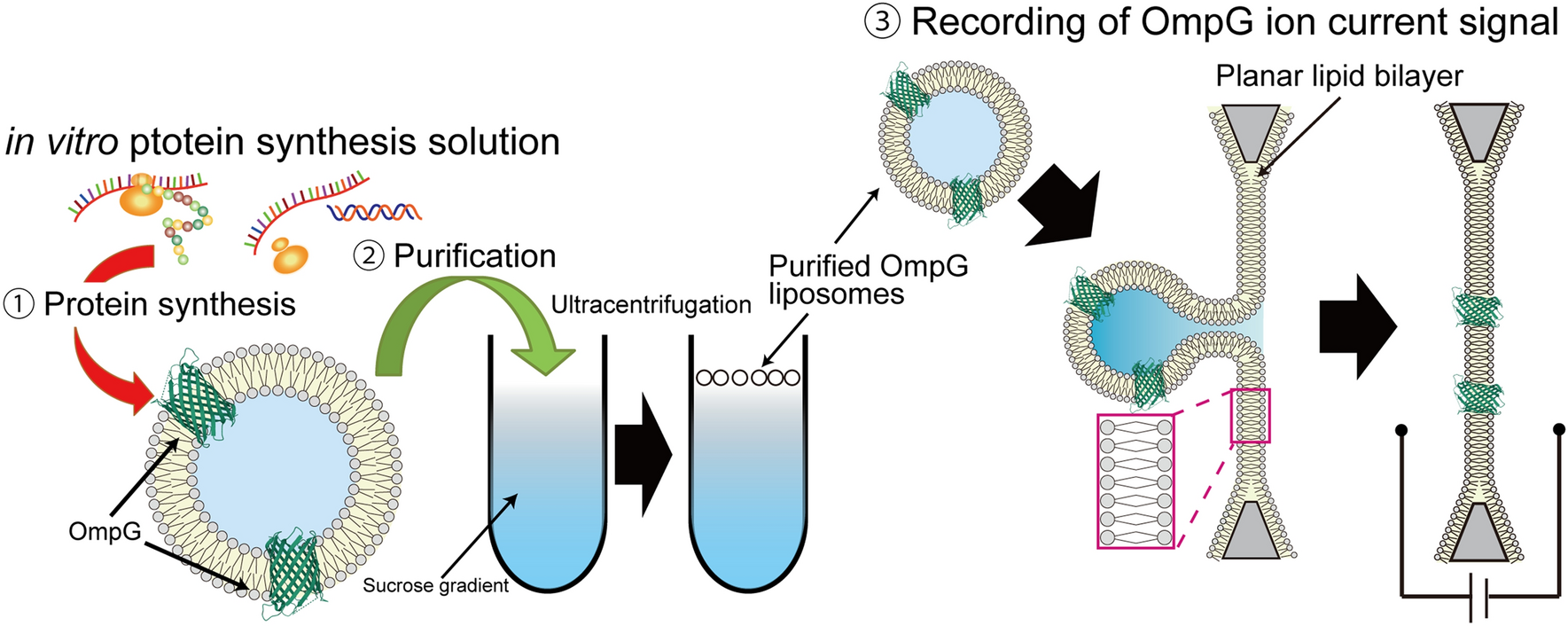The diagram illustrates a detailed step-by-step process of protein synthesis, purification, and recording of OMPG ion current signals. The overall title "In Vitro Protein Synthesis Solution" is prominently displayed at the top in bold text. 

In Step 1, labeled "Protein Synthesis," there is a depiction of a doughnut-shaped structure with outer gray balls and a beige interior, connected by black lines. This structure has a blue interior and is surrounded by green netting with an arrow labeled "OMPG" pointing to Step 2.

Step 2, titled "Purification," features a green arrow directing towards a series of beakers illustrated with black lines and blue interiors, and specifically shows a test tube labeled "Sucrose Gradient" filled with blue and gray liquid. An accompanying green arrow marks the process of "Ultracentrifugation," leading to the label "Purified OMPG Liposomes" with small circles depicted nearby.

Step 3 is marked as "Recording of OMPG Ion Current Signals" and includes an illustration described as planar lipid bilayers. There are two elongated, snake-like chains situated next to each other, indicating the arrangement of proteins in this state. A beige chain with white lines and outer gray balls, fractured by triangular shapes, further elaborates on the structural complexity in this step.

Overall, the diagram visually explains the biological process of protein synthesis and successive steps involved in purifying and recording ion current signals, despite possible typographical errors in the labels.